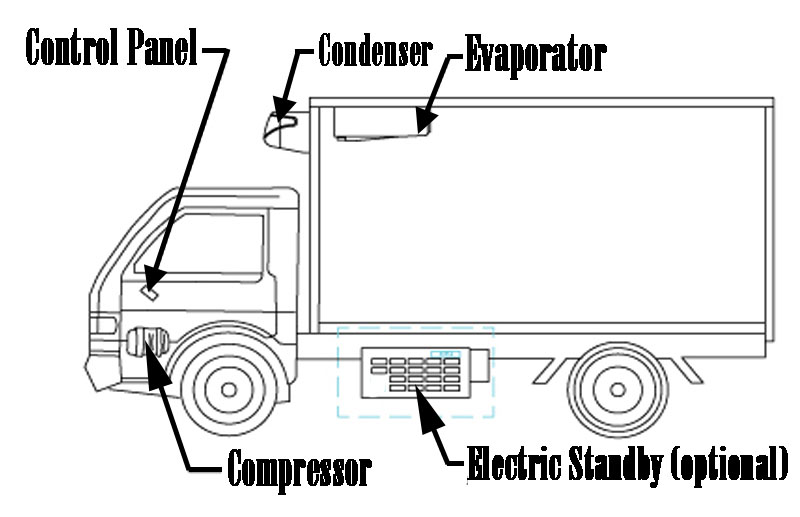The image is a black and white line drawing of a truck in landscape mode, facing towards the left, with various parts labeled through text and arrows. The truck's cab features a title "Control Panel," marked by an arrow pointing down towards the driver's side door area. Just below, another arrow points up to the "Compressor," depicted as a beehive-like structure. The back of the truck includes a large rectangular box representing the cargo area. On the top of this box, arrows point down to the "Condenser" and "Evaporator." Additionally, at the bottom of the cargo box, another arrow points up to the "Electric Standby (Optional)," indicated as a small box with buttons on the other side. The truck is shown with two front wheels and two rear wheels, illustrated using concentric circles. The entire diagram is composed of simple shapes and lines, with all text written in bold black font accompanied by black arrows pointing to each corresponding part.